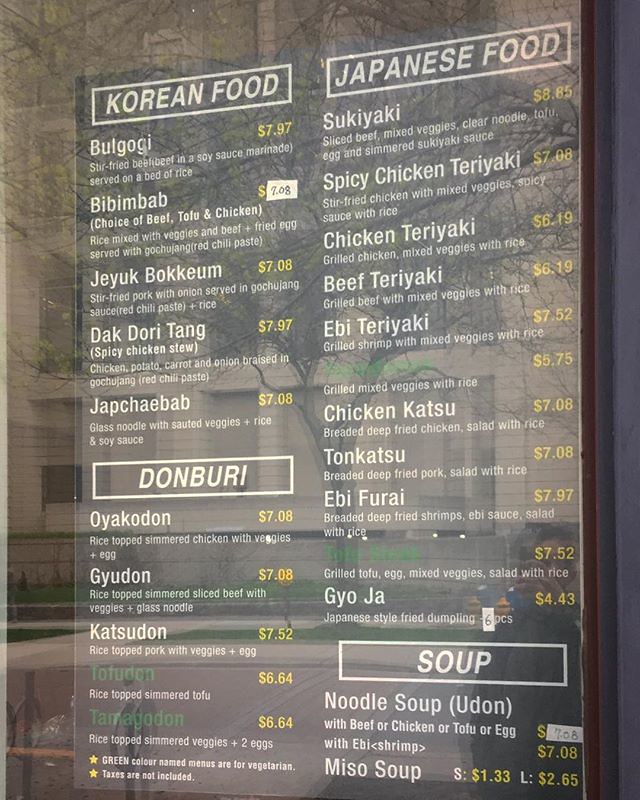Here's a cleaned-up and detailed caption for the image:

---

This is a portrait-style image capturing a restaurant menu through a glass window. The menu prominently features a black background with white text, while the prices are highlighted in yellow. At the top, a section framed by a white outline reads "Korean Food."

1. **Bulgogi - $7.97**: Stir-fried beef marinated in soy sauce, served on a bed of rice.
2. **Bibimbap - $7.08**: Choice of beef, tofu, or chicken mixed with rice, vegetables, and topped with a fried egg, served with gochujang (red chili paste).
3. **Jeyuk Bokkeum - $7.08**: Stir-fried pork with onions, served in gochujang sauce with rice.
4. **Dakdoritang - $7.97**: Spicy chicken stew with potatoes, carrots, and onions, braised in gochujang.
5. **Japchae Bap - $7.08**: Glass noodles with sautéed vegetables, rice, and soy sauce.

Beneath this section, another white rectangle outlines the "Donburi" options:

1. **Oyakodon - $7.08**: Rice topped with simmered chicken, vegetables, and egg.
2. **Gyudon - $7.08**: Rice topped with simmered beef, vegetables, and glass noodles.
3. **Katsudon - $7.52**: Rice topped with pork, vegetables, and egg.
4. **Tofudon (green font) - $6.64**: Rice topped with simmered tofu.
5. **Tamagonidon - $6.64**: Rice topped with simmered eggs.

In the top right corner, contained within a white box, is a section labeled "Japanese Food" which lists:

- Chicken Teriyaki
- Beef Teriyaki
- Yubi Teriyaki
- Spicy Chicken Teriyaki
- Chicken Katsu
- Tonkatsu
- Yubi Furai
- Gyoza

All items are priced within the $6.00 to $7.00 range.

The bottom right corner of the menu details a selection of soups, including noodle soup and miso soup, within a white rectangle labeled "Soup."

---